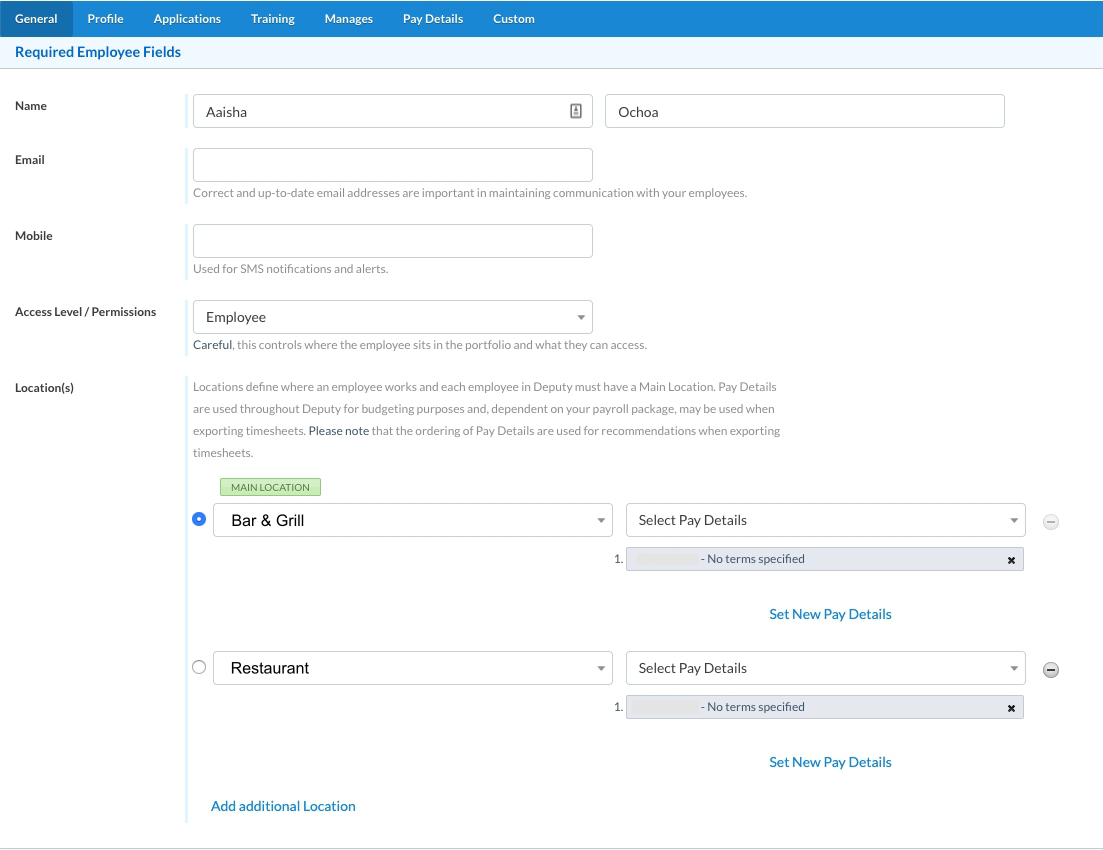This is a comprehensive screenshot of what appears to be an HR system interface. At the very top, a blue banner spans the screen, featuring white links to various tabs. The first tab, “General,” is highlighted in a darker blue, indicating it's the selected tab. To its right are the tabs: Profile, Applications, Training, Manages, Paid Details, and Custom.

Beneath the banner, on a light blue or gray background, is a header in blue that reads "Required Employee Fields." A gray line break demarcates this section from the white background below.

On the left side of the white background, "Name" is written in dark gray, accompanied by a blue line on the right. Two text boxes follow: the first contains the name "AISHA," and the second "OCHOA," likely indicating the first and last names, respectively. Below the name section is the "Email" label in dark gray with the corresponding blue line, followed by an empty text box. Underneath the email text box, in gray text, it says "Correct and Up-to-Date. Email addresses are important in maintaining communication with your employees."

Similarly, under the "Email" section is "Mobile," with the familiar blue line and a blank text box next to it. Beneath this, it reads, "Use for SMS Notifications and Alerts."

Next is the "Access Levels/Permissions" section in gray text with a blue line to its right. A drop-down menu reads "Employee" in dark gray. Below this, bolded in dark gray, it says "careful," followed by non-bolded text explaining, "This controls where the employee sits in the portfolio and what they can access."

The "Locations (s)" section follows, with explanatory text in gray: "Locations define where an employee works, and each employee and deputy must have a main location. Pay details are used throughout deputy for budgeting purposes and, depending on your payroll package, may be used when exporting timesheets." A note in bluish gray and bold text says, "Please note," followed by, "that the ordering of pay details are used for recommendations when exporting timesheets."

There are two location options displayed. The top option includes a filled blue radio button with a drop-down menu that says, "Bar & Grill." A green badge labeled "Main Location" stands out, paired with an unselected drop-down menu for "Select Pay Details" and a collapsible button symbolized by a gray circle with a line. Below it, “1” is indicated in dark gray, followed by yellow text on a gray background (illegible), "No Terms Specified," and an “X” to the right. A blue link below says, "Set New Pay Details."

The second location option has an empty radio button and a drop-down menu that has "Restaurant" selected. To the right, similar to the top option, it says "Select Pay Details" with the same collapsible button. Below this, it again shows "1," "No Terms Specified," and an "X," followed by "Set New Pay Details."

Finally, at the bottom left, in blue text, is "Set New Pay Details, Add Additional Location."